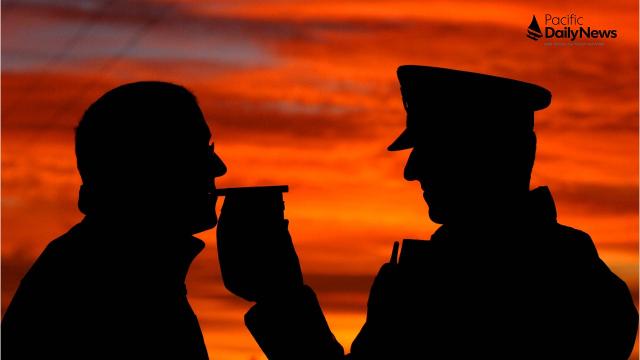In this slightly blurred, silhouetted image, two figures stand against a soft-focus, fiery sunset dominated by hues of gold, orange, and red. Positioned to the left is the silhouette of a man, his hair likely reaching his collar and possibly wearing glasses. Opposite him, on the right, is another man in a military or captain's hat, distinguished by the silhouette of insignias or medals on his uniform. This right-side figure holds an object near the other man's mouth—perhaps a cigarette or similar item. The overall composition suggests an advertorial for Pacific Daily News, whose logo appears in the top right corner of the image. The format of the image is notably longer than it is tall.